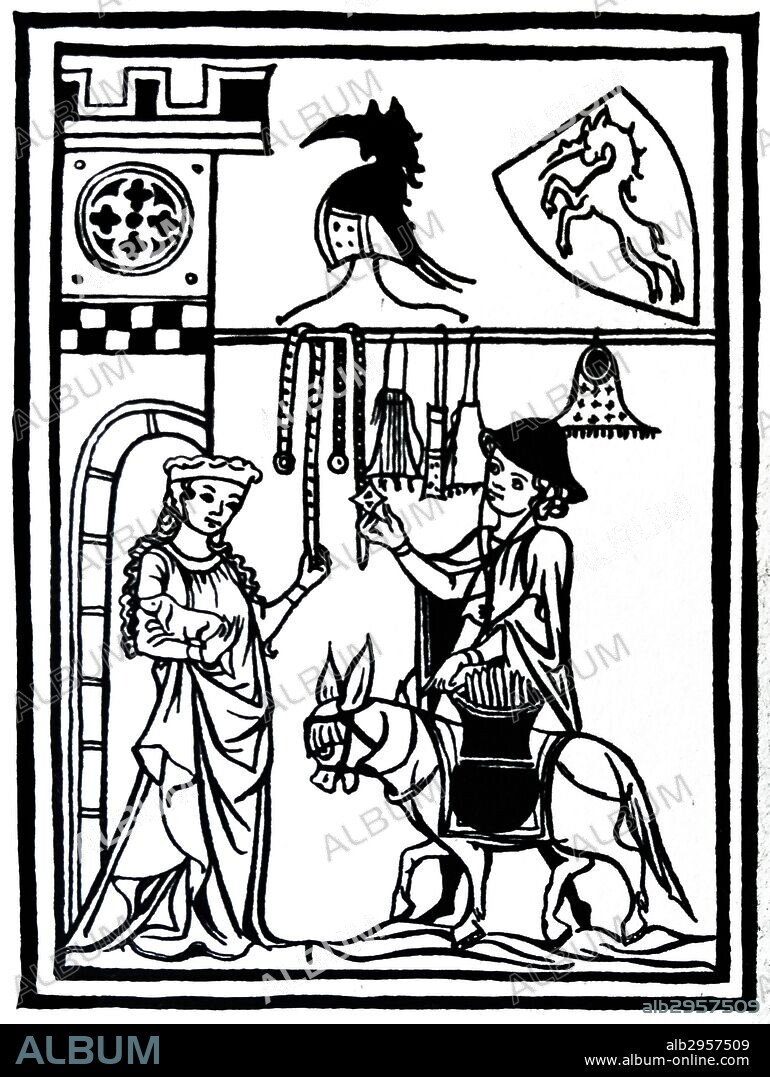The black and white illustration titled "Album" at the bottom in blue letters is a detailed depiction of a scene reminiscent of the 1800s or an older European era, possibly set in a location like France or Germany. It portrays a castle gate with an intricately shaded black wall in the background, giving the scene a medieval ambiance. To the left stands a regal princess, adorned in a finely detailed dress and a crown, signifying her royal status. She holds a small puppy in her right arm while examining a pole laden with a variety of wares, which includes ropes, belts, and possibly weapons or tools, suggesting the man next to her—dressed simply and accompanied by a donkey—is a merchant showcasing his goods. A bell hangs prominently, and a shield featuring a horse or unicorn emblem adds to the imagery of chivalry and medieval life. The overall scene is meticulously outlined in thin black lines, with larger objects filled in with darker shades, enhancing the picture's depth and historical texture.